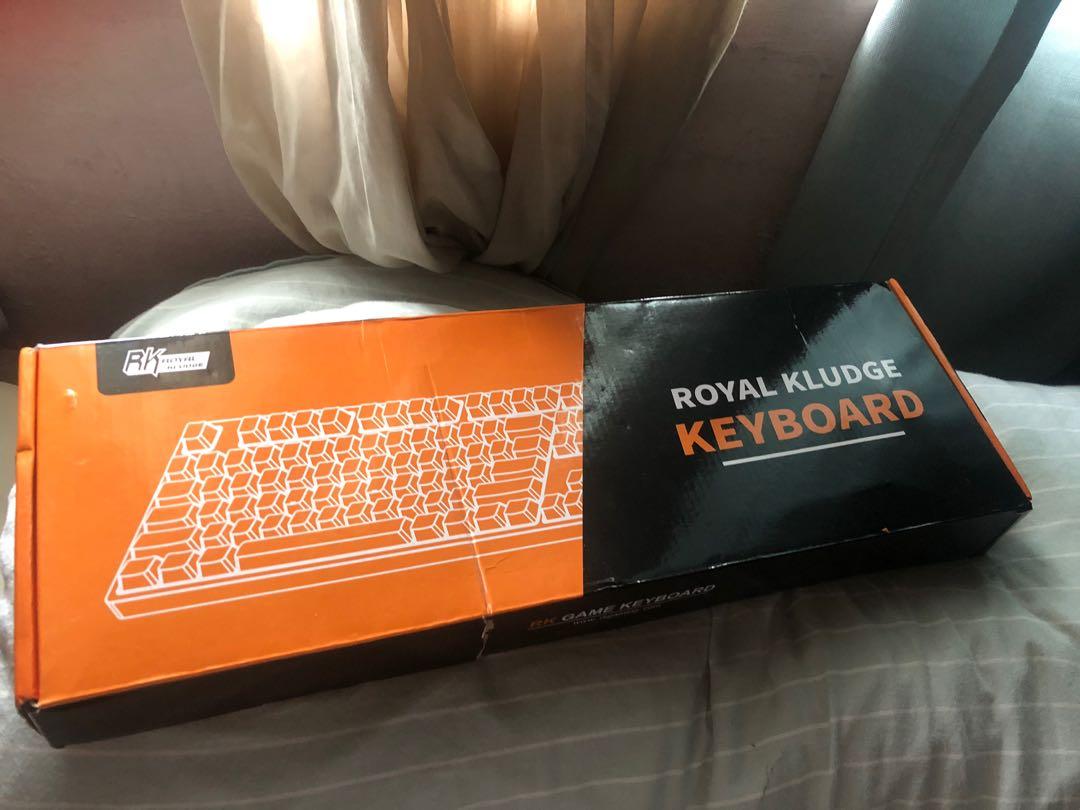The image reveals a detailed scene centered around a boxed keyboard. The keyboard rests atop what appears to be a grayish blanket adorned with white stripes, suggesting a bed as its base. In the soft background, translucent beige curtains allow sunlight to filter through, indicating that the photograph was taken during the daytime. The walls of the room have a subtle pinkish hue, adding a warm tone to the overall ambiance.

The primary focus of the photo is the keyboard displayed in its packaging. The box is distinctly divided: the left half is a vibrant orange, while the right half is a sleek black. The black section features the brand name "Royal Kludge" in white text and the word "Keyboard" in an orange font, creating a visually appealing contrast. On the left orange section, a partial image of the keyboard is visible, showcasing its design. The keyboard itself is outlined in white, with orange keys that stand out boldly. Additionally, the top of the box displays a black label with the initials "RK." Some text is also visible along the sides of the box, providing further details about the product contained within.